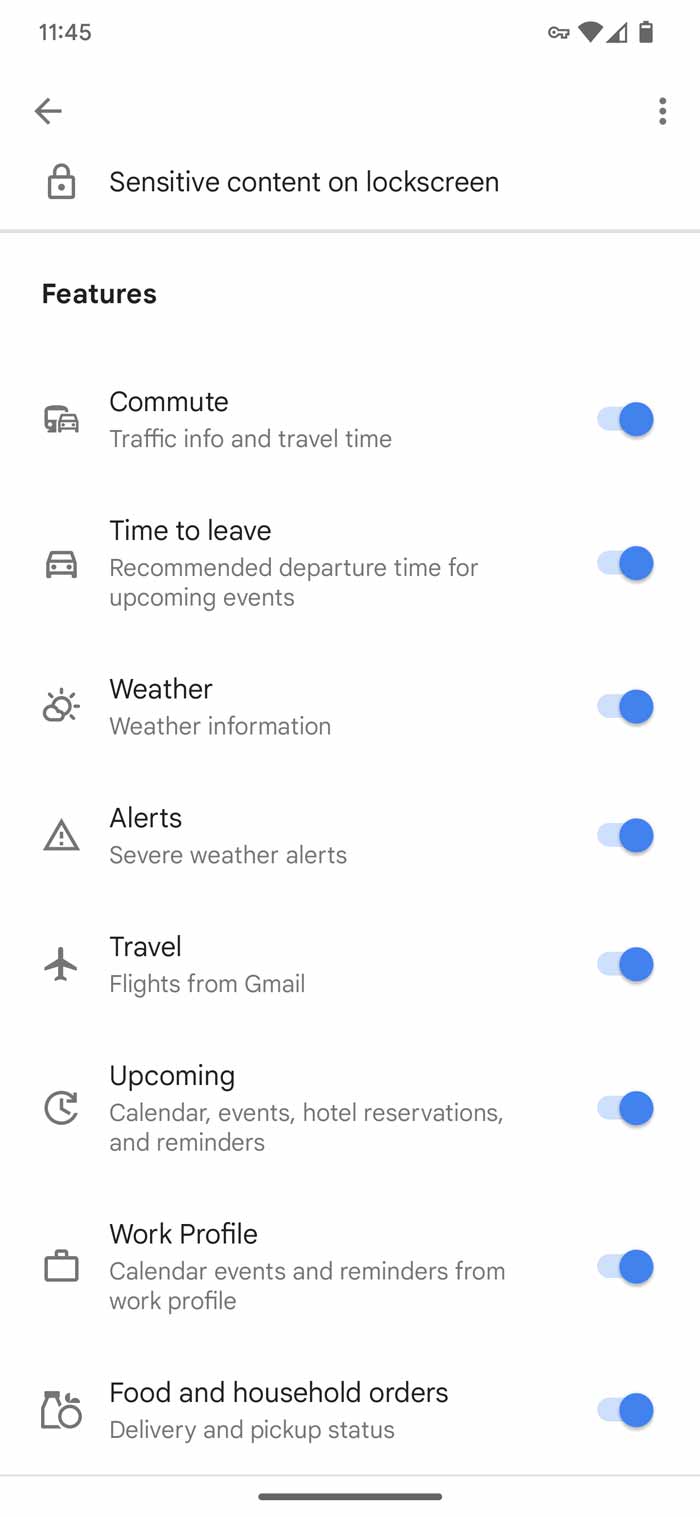This is a detailed screenshot of a mobile device's notification settings, showcasing various features being configured. The time displayed is 11:45, and the top-right corner features status icons for a key symbol, Wi-Fi connection, data signal strength, and battery life, which appears to be at around 80-90% capacity. Just below the information bar, a notification reads "Sensitive content on lock screen."

Underneath, there's a heading labeled "Features." Below this are several features listed vertically, all of which are currently enabled as indicated by the toggles being switched to the right and highlighted in blue.

The listed features and their corresponding icons are as follows:
1. **Commute** 
2. **Traffic info and travel time**
3. **Time to leave**
4. **Recommended departure time for upcoming events**
5. **Weather Information**
6. **Severe weather alerts**
7. **Flights from Gmail**
8. **Calendar events, hotel reservations, and reminders**
9. **Events and reminders from work profile**
10. **Delivery and pickup status**

The layout and organization of the settings imply a high level of customization and attention to detail, ensuring that the user receives all relevant notifications in a timely and organized manner.